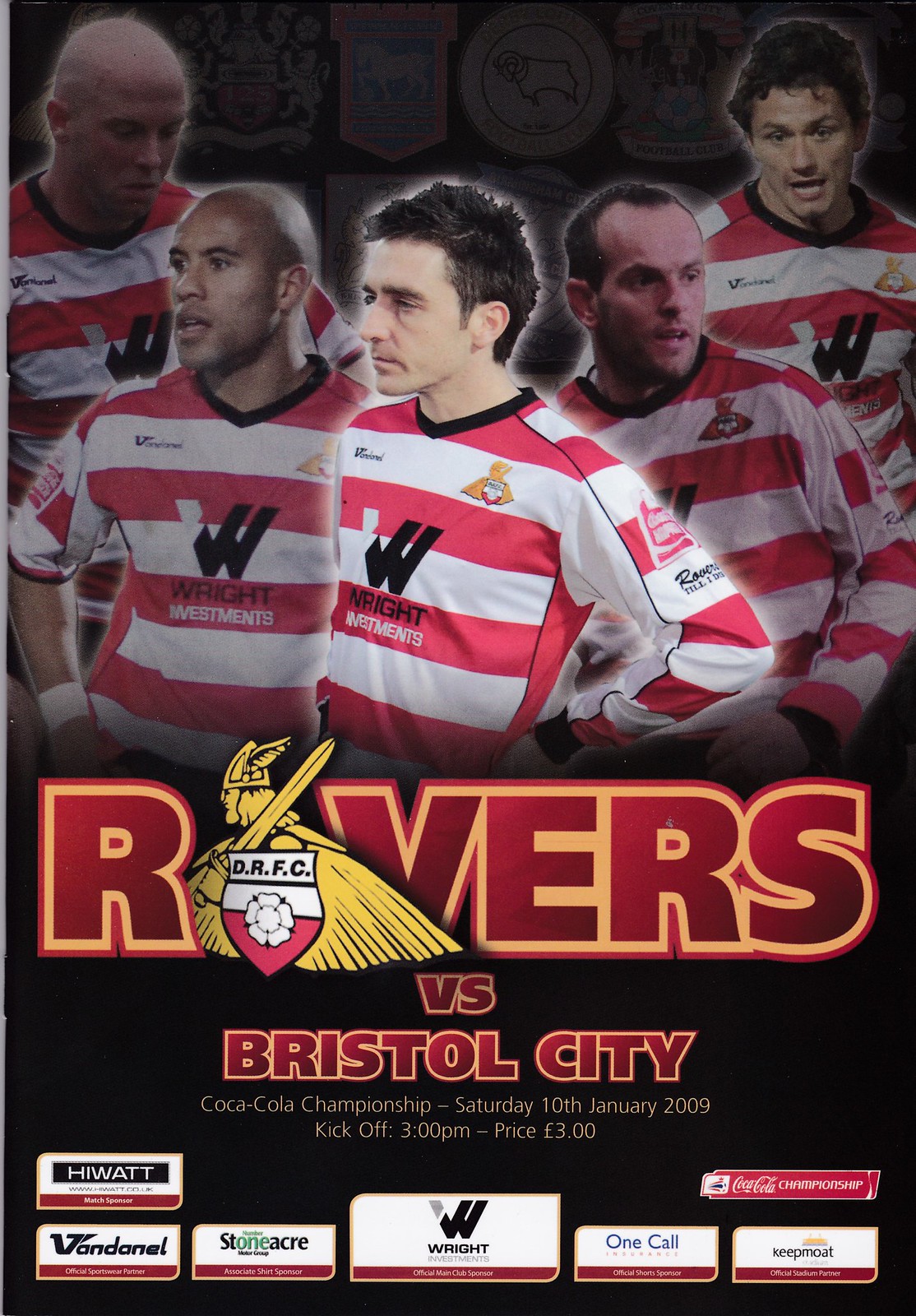The image is an advertisement or flyer for a football match featuring the Rovers Football Club. At the top, there is a full-color photograph of five football players dressed in identical kits: white and red striped shirts with black collars, emblazoned with the "Bright Investments" logo featuring a prominent black "W." Below the players, the word "Rovers" is displayed in bold red font with an orange border, where the "O" is replaced by a Viking logo facing left. Beneath this, red text announces the match details: "Rovers vs Bristol City," followed by "Coca-Cola Championship, Saturday, 10th January 2009, kickoff 3 p.m." The ticket price is listed as "3 pounds" in yellow font. At the very bottom, there are multiple rectangles showcasing various business logos, suggesting the sponsors of the event, including companies like Wright, Stone Acre, HeWatt, OneCall, KeepMote, and Coca-Cola. The overall design appears to be for an English soccer match program, with the players centrally positioned, creating a visually engaging composition that emphasizes the upcoming event and its sponsors.